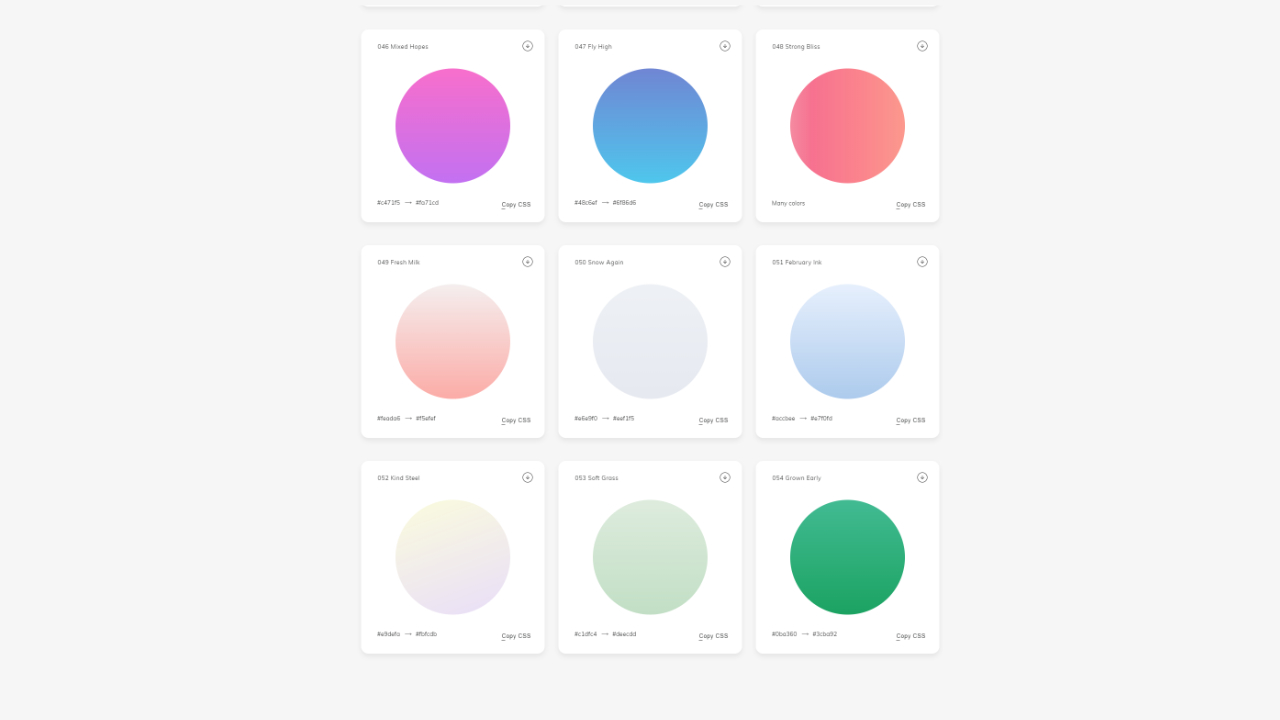This image features nine square white tiles arranged in a 3x3 grid against a light gray background. Each tile contains black text in the upper left corner, with a symbol in the upper right corner, and additional writing in both the bottom left and right corners. The tiles are positioned centrally within the gray backdrop. The circles on the tiles exhibit a variety of colors, distributed as follows: the top row showcases a pink circle, a blue circle, and a reddish peach circle. The middle row features a blended peach and white circle, a light smoke-gray circle, and a bluish-gray circle. The bottom row includes a lavender and yellow circle, a green and white circle, and a solid green circle, from left to right.